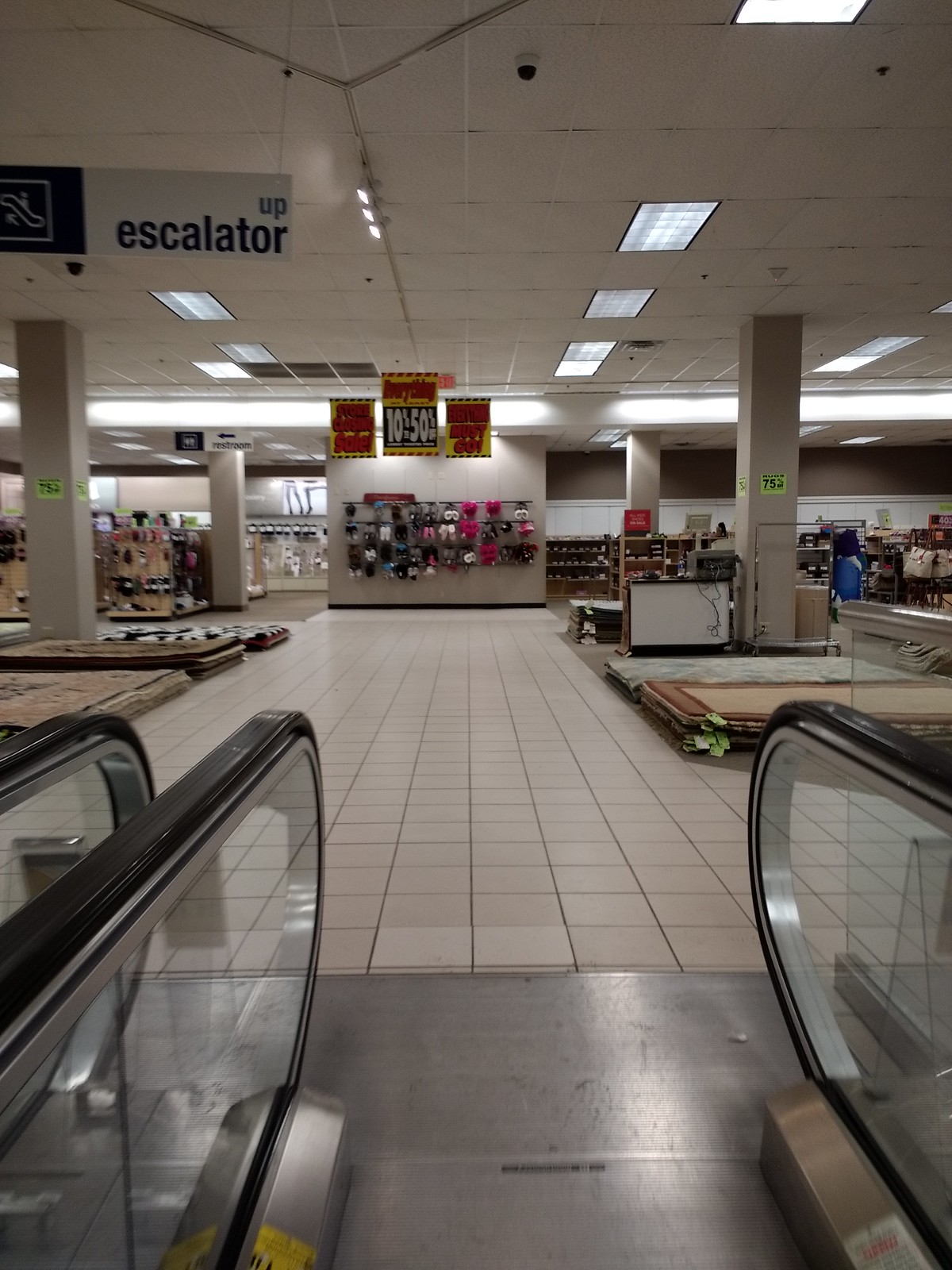The photograph captures the interior of a department store, viewed from the perspective of someone ascending an escalator. The escalator's rails and steps are prominently visible in the foreground. As one steps off the escalator onto white flooring, various piles of area rugs with price tags and descriptions immediately come into view. The store appears to be in the midst of a going out of business sale, evident from the significant "75% off" signs displayed on thick square pillars scattered throughout the area. 

In the mid-ground, there is a cashier's area situated close to the rug displays. The ceiling is lined with acoustic tiles, contributing to the store's ambiance. 

In the distant background, another set of sales displays is visible, showcasing numerous slippers and tennis shoes hung on rails beneath a board that proclaims "Everything 10-50% off, all sales final." Signs hanging from the ceiling reiterate this discount. To the left of the shoe display, there are additional racks of shoes and socks, though they are small and somewhat difficult to distinguish. To the right, accessories such as handbags are arranged, adding to the variety of discounted items available in this closing sale.